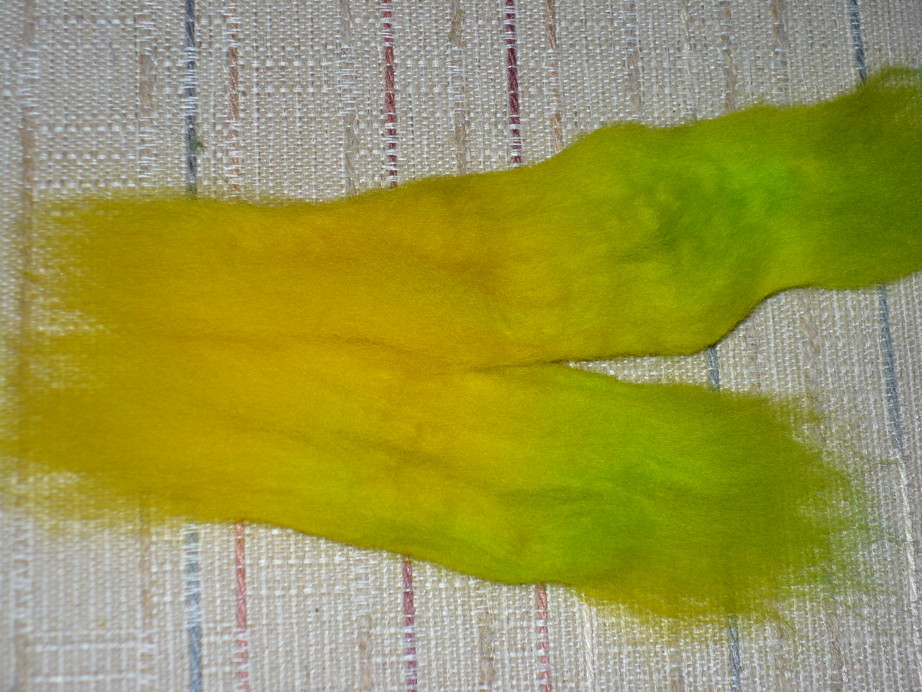The image displays a yellow and green fabric or wispy material, resembling hair or perhaps a scarf, which stretches horizontally across the foreground. It starts as bright yellow on the left and gradually transitions into green as it extends to the right. This material appears to split into two strands, connecting at the top and diverging into a V-shape towards the right. It lies on top of a woven rug featuring a tan and white base with colored vertical stripes. The stripes include shades of blue, red, tan, gray, and pink, repeating in a vertical pattern. The overall scene blends soft textures and vibrant colors, creating a visually intriguing composition.